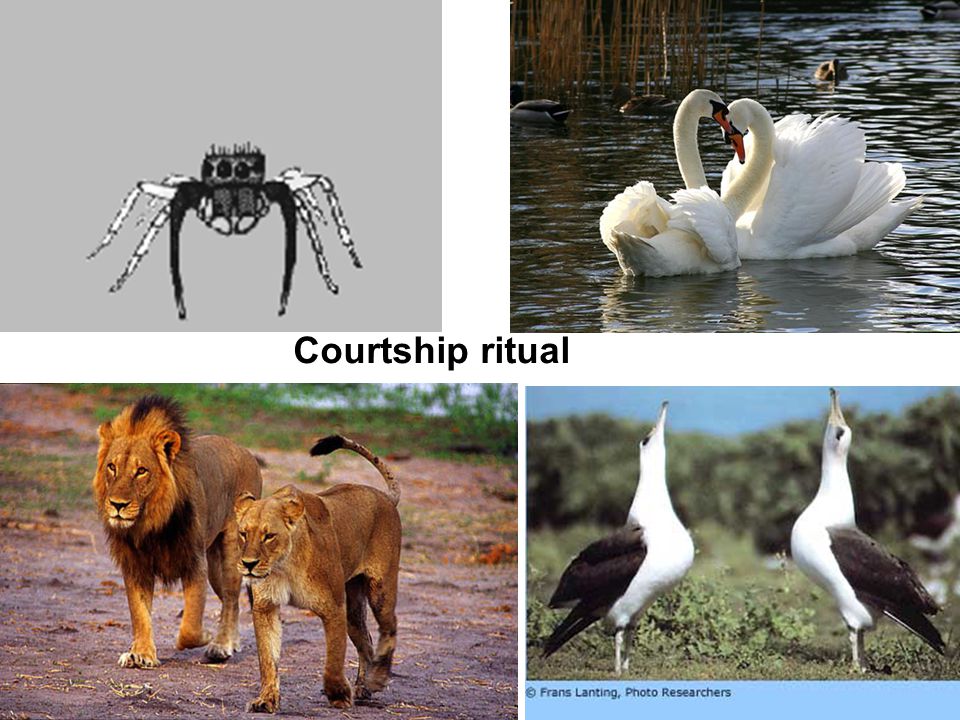The image is a composite of four different pictures, unified under the title "Courtship Ritual" written in black text at the center. In the upper left, there is a black-and-white digital illustration of a spider with a gray background. The spider has large black eyes, black front legs, and white hind legs. In the upper right, two swans are depicted on a glistening body of water, with their heads pressed together to form a heart shape. The lower left shows a photograph of a male and female lion walking on red dirt with small green shrubs in the background; the male lion has a dark mane while the female does not. Finally, the lower right features two birds, resembling pelicans, with white bodies and gray wings, standing in a dirt area with their beaks pointed upward, set against a backdrop of green trees and an open field.